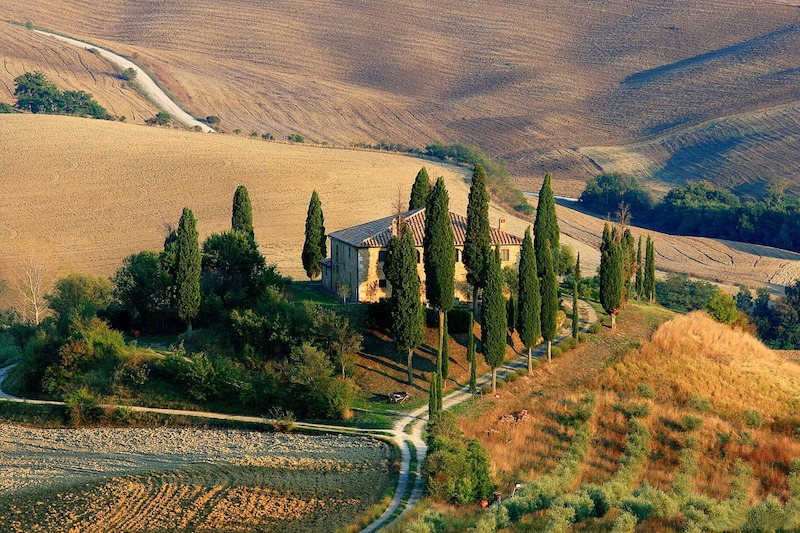This is a detailed color landscape photograph taken from above, possibly by a drone, showcasing a picturesque countryside scene. The central focus is a beige stucco farmhouse with a red tile roof, partly obscured by tall, conical green cypress trees. The farmhouse, seemingly a single-story structure, is situated amidst expansive fields of yellow, brown, and green tones, emphasizing a serene rural setting. 

A narrow, winding road traverses the lower portion of the image, moving from the bottom center, curving right, left, and right again, before disappearing behind the house. To the viewer's right, there's a mix of dense shrubbery and greenery, with a sloping area that transitions from meticulously planted rows to a backdrop of golden, dead grass. Beyond this, the landscape extends into a large valley dotted with fields of similar golden vegetation, underscoring the vast openness of the area. Rolling hills in the distance contribute to the tranquil countryside atmosphere. This representational realism photograph captures the tranquil beauty and vastness of rural life through its rich and natural color palette of greens, yellows, tans, and browns.